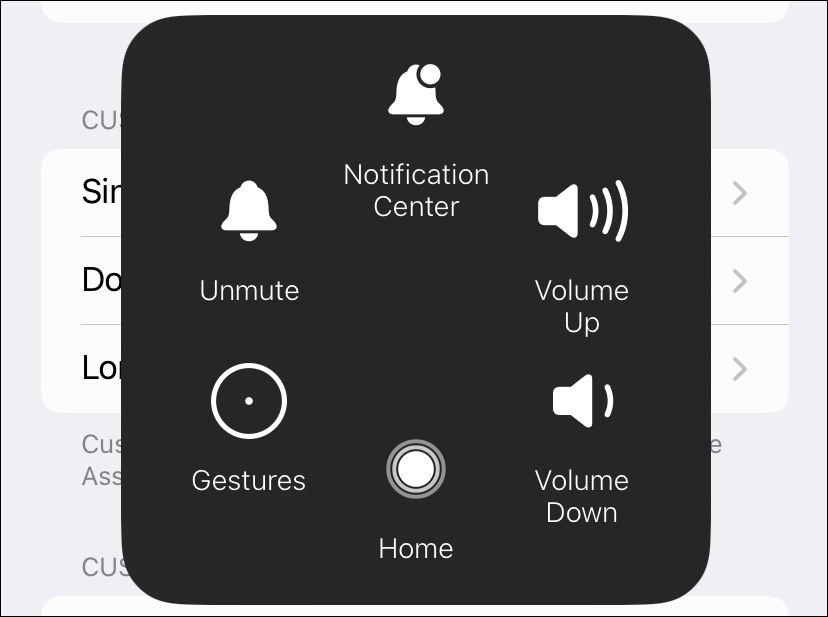The image features a black-outlined rectangle with a gradient gray fill and some text partially obscured by a large black square. At the top of the rectangle, there is a white section. Though the text under the black square is mostly illegible, a few elements are visible on the right-hand side: three right-pointing arrows, separated by gray lines, each within a white square. The top square has a curved upper right corner, and the bottom square has a curved lower right corner.

Inside the large black square, the text "Notification Center" is prominently displayed at the top, accompanied by an icon of a bell with a small circle above it. On the left side of the black square, there is another bell icon labeled "Unmute." Below that, a speaker icon with sound waves is labeled "Volume Up." There is also a white circle with a smaller white dot in the center, labeled "Gestures." Further down, a gray and lighter gray outlined circle with a white center is labeled "Home." Lastly, another speaker icon with a single sound wave is labeled "Volume Down."